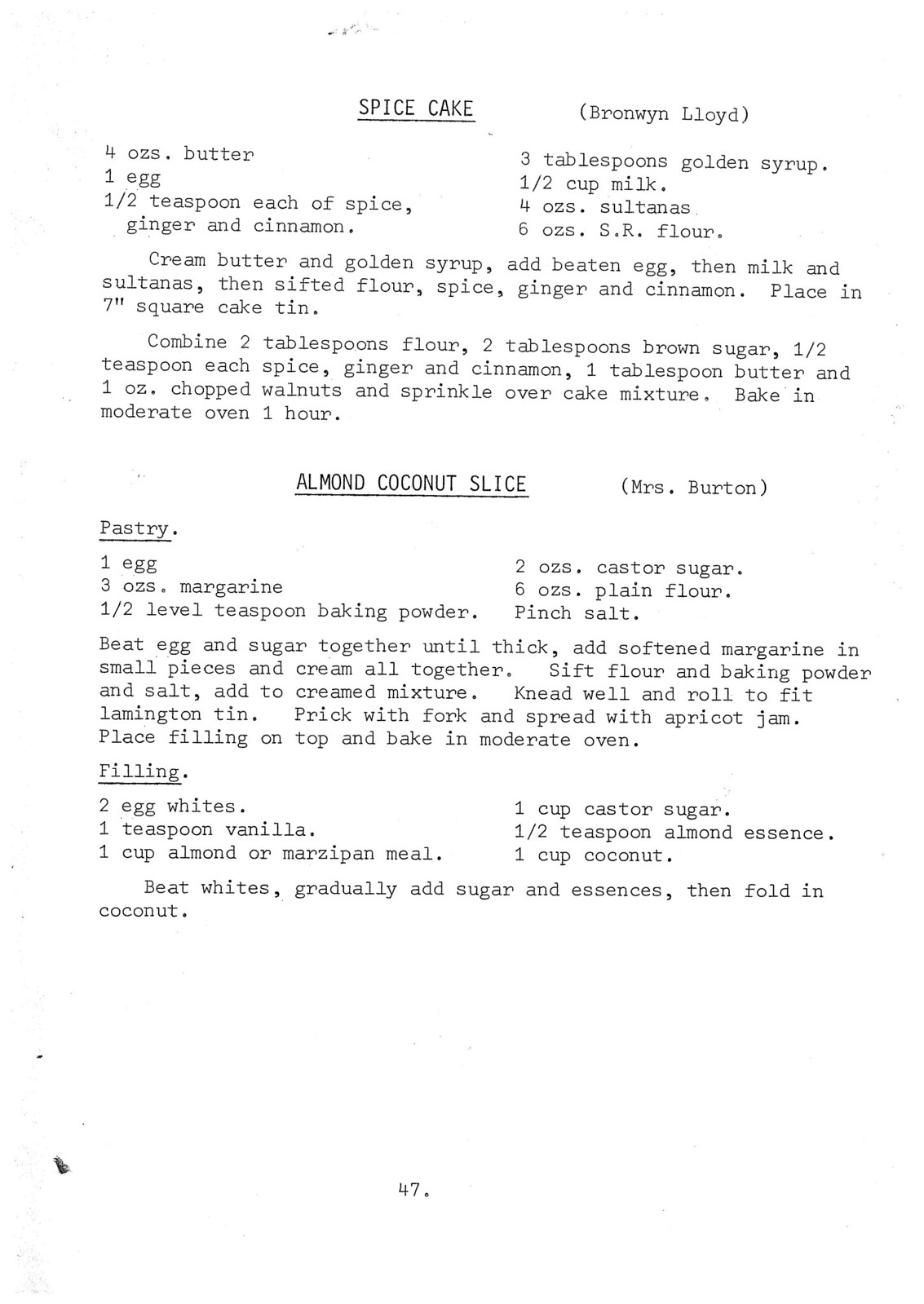This image, printed in black type on white paper, features a detailed, typewriter-style recipe for Spice Cake by Bronwyn Lloyd. The recipe begins with four ounces of butter, three tablespoons of golden syrup, one egg, and a half cup of milk. It calls for a half teaspoon each of spice, ginger, and cinnamon, four ounces of sultanas, and six ounces of self-raising flour. The instructions detail creaming the butter and golden syrup, adding a beaten egg, then the milk and sultanas, and finally sifting and mixing in the flour, spice, ginger, and cinnamon. The mixture is to be placed in a seven-inch square cake tin. A topping is made by combining two tablespoons of flour, two tablespoons of brown sugar, a half teaspoon each of spice, ginger, and cinnamon, one tablespoon of butter, and one ounce of chopped walnuts, which is sprinkled over the cake mixture. The cake is baked in a moderate oven for one hour. Below this recipe is another for Almond Coconut Slice by Mrs. Burton, containing similar ingredient lists and instructions. The page concludes with the number 47 at the bottom.